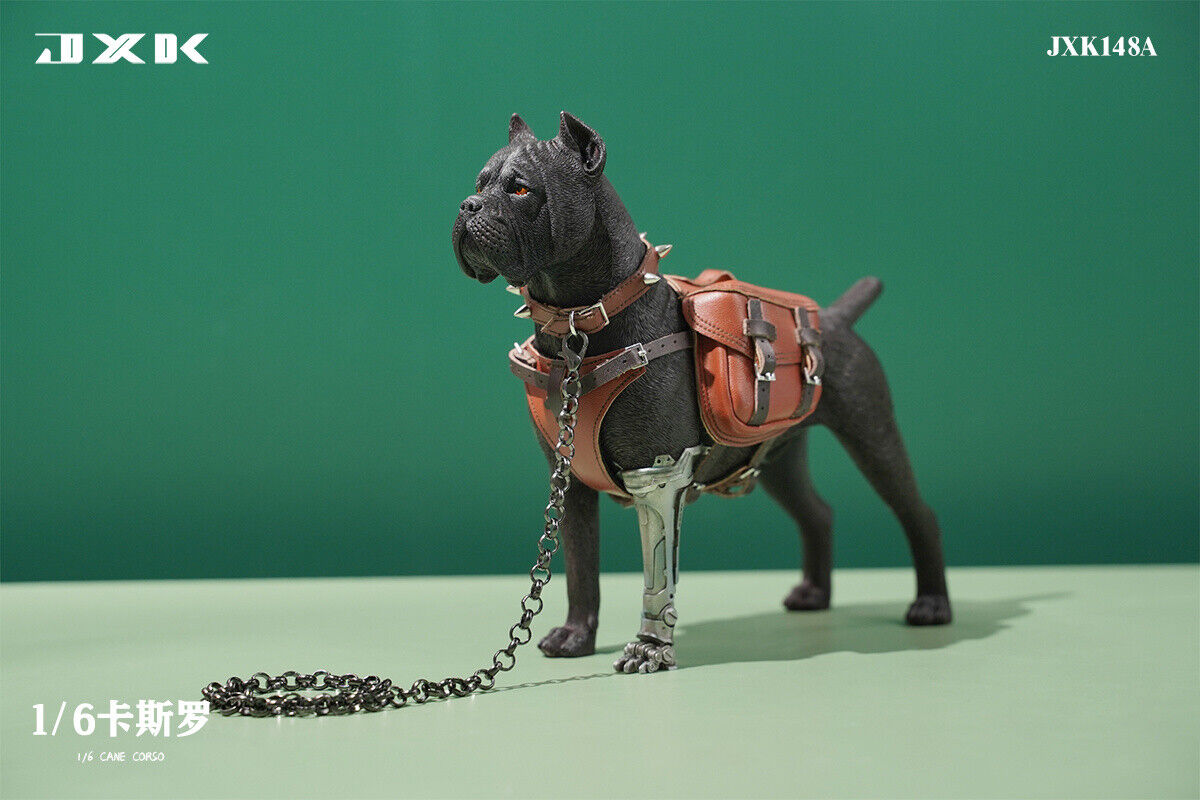This detailed photograph captures a 3D figurine of a Cane Corso or pit bull-style dog, meticulously rendered in a blend of realistic and artistic elements. The focal point is the dog standing proud at the center, its left front leg replaced by a Terminator-esque robotic limb, showcasing a metallic exoskeleton. This hybrid aesthetic is further enhanced by a brown leather vest draped across its chest and back, paired with a matching leather saddlebag. The dog is decorated with a spiked brown leather collar, from which a chain leash extends and coils on the surface beneath it. The dog's light brown eyes gaze to the left, complementing its robust and vigilant stance.

The figurine rests on a light beige or seafoam green table, which contrasts with the solid dark green background. In the top left corner, the white lettering "JXK" is displayed in an artistic font, while the top right corner reads "JXK-148A." In the bottom left, there are small, intricate Japanese characters along with the number "1-6." This scene encapsulates a fusion of traditional craftsmanship and modern robotic aesthetics, providing a compelling visual narrative.